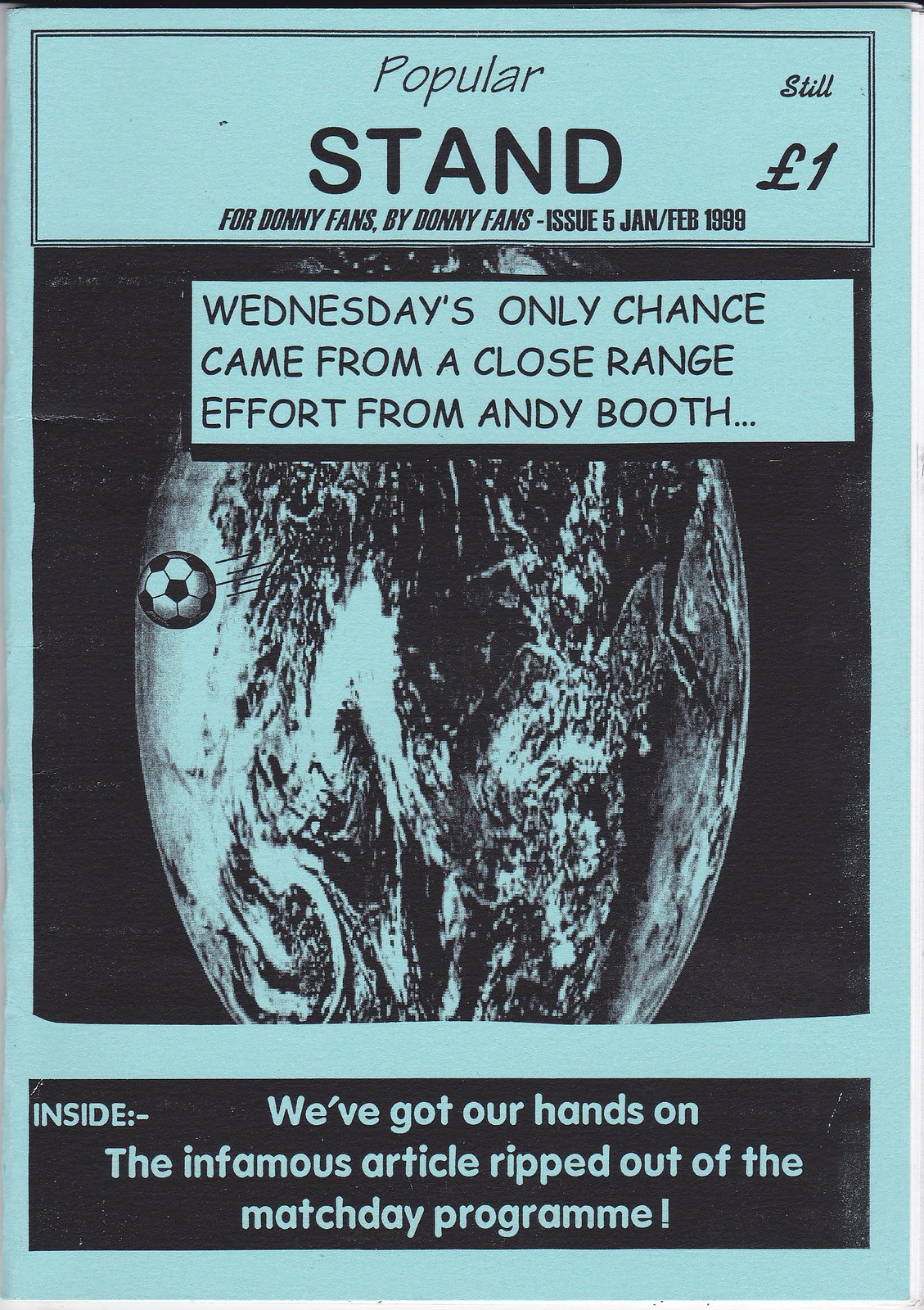The image depicts the cover of a magazine titled "Popular Stand" in pale blue and black hues. At the top, it reads, "For Donnie Fans, By Donnie Fans, Issue 5, January-February 1999, Still One Pound." The price is denoted with the British pound symbol (£). Beneath this, a black box contains the text: "Inside: We've got our hands on the infamous article ripped out of the Match Day program!" Centrally, there is a vertically stretched black-and-white image of the Earth, with a soccer ball emerging from it. Additional text on the cover mentions, "Wednesday's only chance came from a close-range effort from Andy Booth." The design includes black borders at the top and along the edges of the cover.